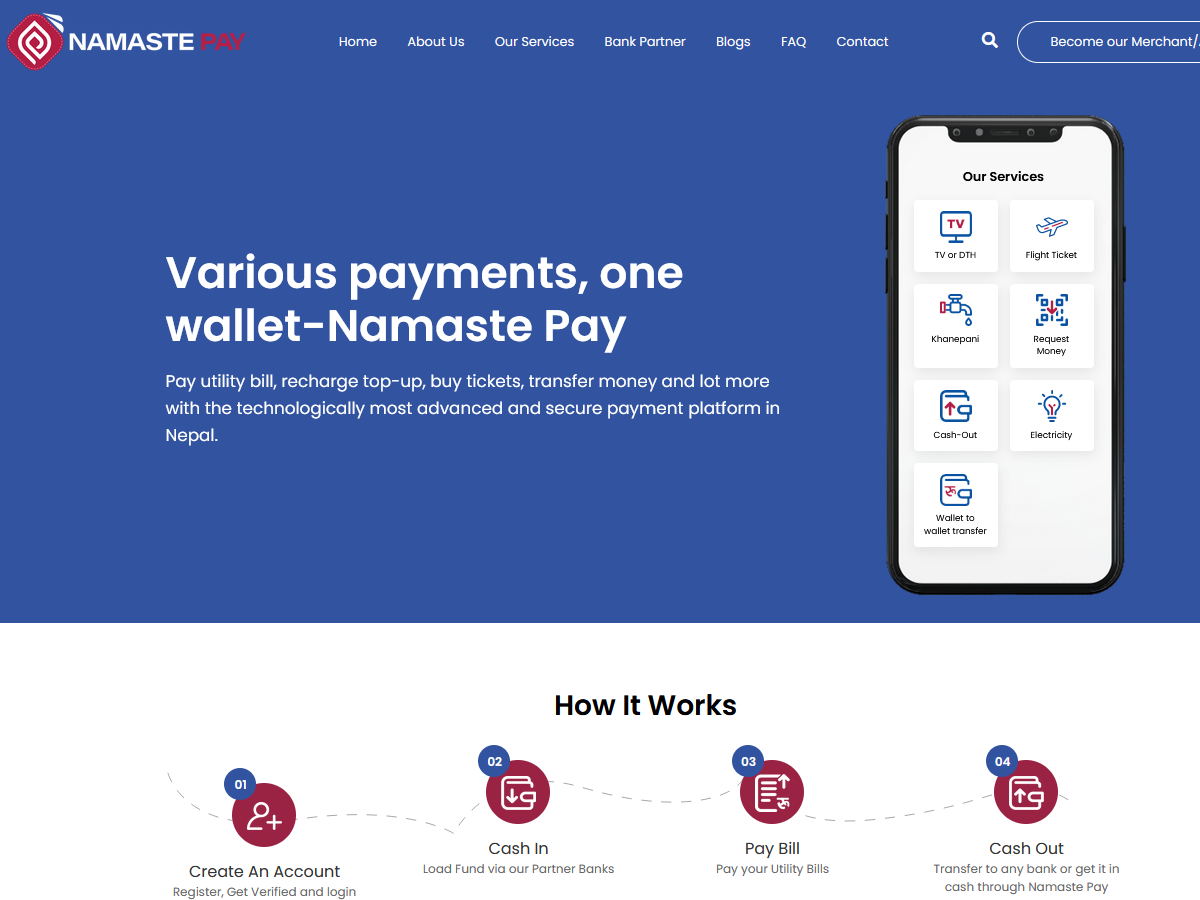The image showcases the NamastePay website interface prominently. At the top of the webpage, a navigation bar is visible featuring the categories: Home, About Us, Our Services, Bank Partners, Blogs, Facts, and Contact. A search bar is positioned on the side of the page for user convenience.

The main content area highlights various payment functionalities offered by NamastePay, described as one of the most technologically advanced and secure payment platforms in Nepal. The available services include utility bill payments, phone recharges, top-ups, ticket purchases, and money transfers, among others.

On the right side of the webpage, an illustration of a phone displays these services in more detail. Categories such as TV recharges, flight tickets, company requests, monthly payments, cash queues, electricity payments, and more are represented by icons. However, some text is difficult to read due to the small font size.

A step-by-step guide titled "How It Works" is also visible, outlining the process for users: first, create an account, then cash in, proceed to pay bills, and finally, cash out. The design and layout aim to simplify the user experience while providing comprehensive payment solutions.

Overall, the NamastePay website is depicted as a versatile and secure platform for managing various financial transactions in Nepal.